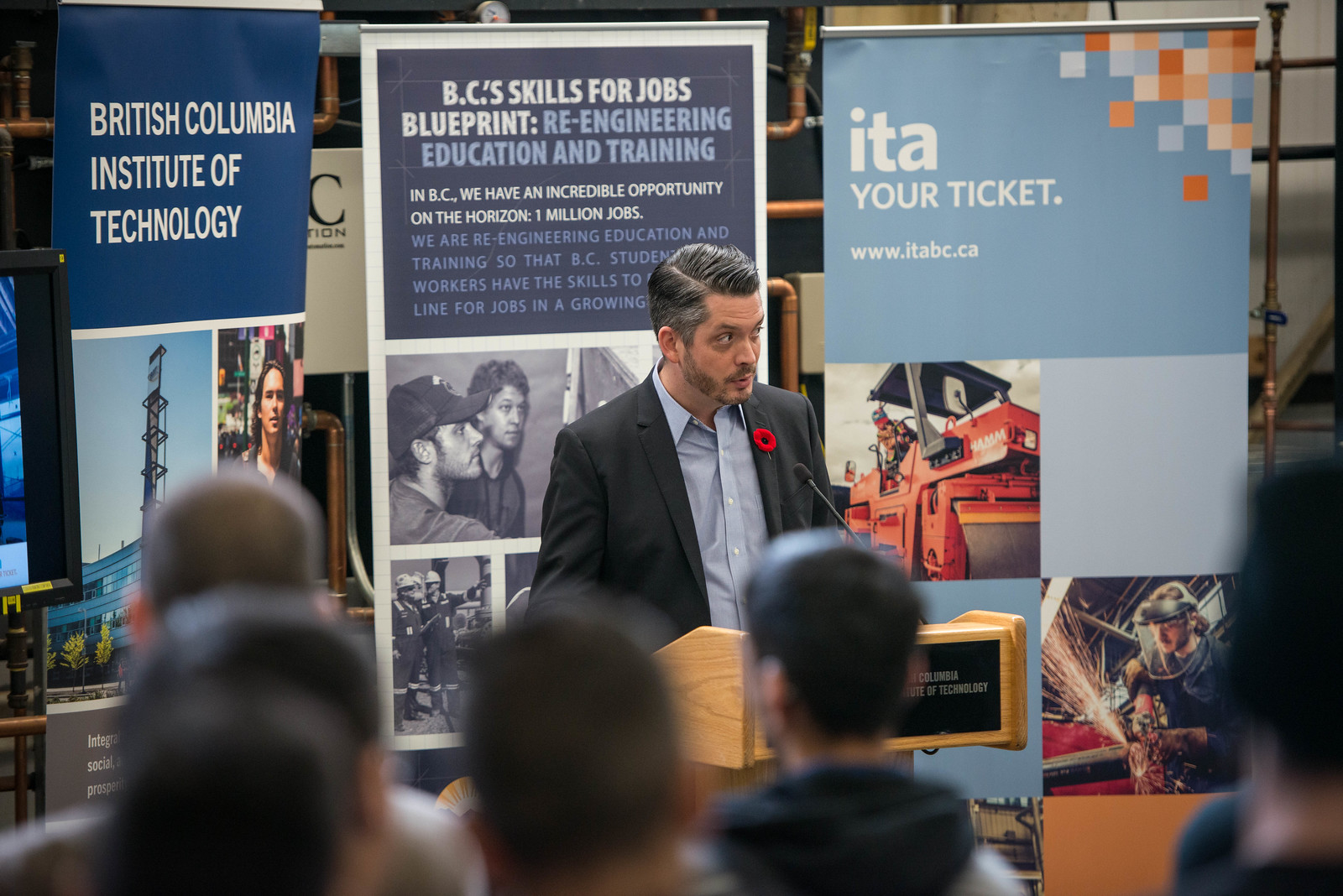A distinguished gentleman with neatly combed gray hair, dressed in a suit without a tie, stands at a wooden podium, addressing an audience. He dons a red circular pin on his lapel and speaks into a microphone positioned about six inches from his face. Behind him are three blue banners; the one on the left reads "British Columbia Institute of Technology," the center banner states "BC Skills for Jobs Blueprint: Re-engineering Education and Training. In BC we have an incredible opportunity on the horizon: 1 million jobs. We are re-engineering education and training so that BC student workers have the skills in line for jobs in a growing world," and the one on the right says "ITA, your ticket." The audience members, though blurred in the photo, are attentive, with at least seven visible from the back. The setting appears to be an indoor seminar or presentation, with the large horizontal rectangular image capturing both the speaker and his message-focused backdrop.